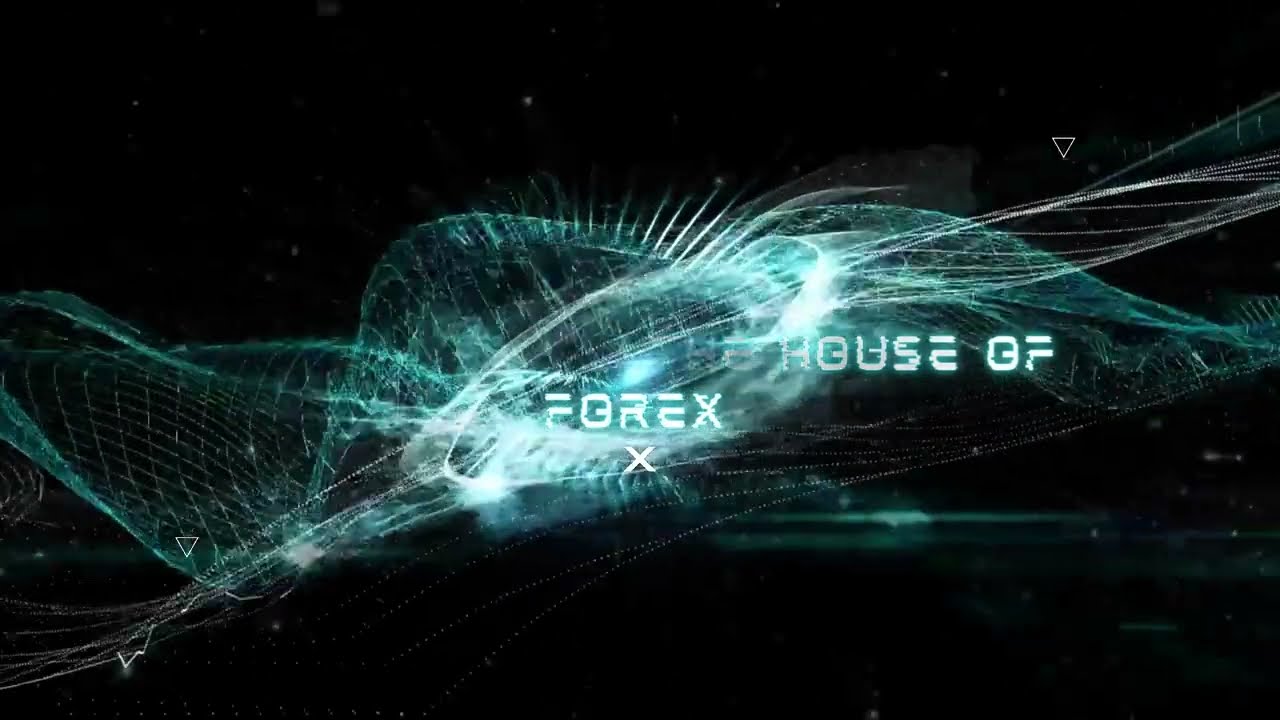The image features a complex and computer-generated design set against a completely black background. Dominating the center, the design appears as a detailed, 3D spiral or wave pattern that encompasses various geometric shapes such as triangles and squares, laid out in a checkerboard-like arrangement. The spiral extends diagonally from the bottom left to the upper right corner and is rendered in hues of light blue, green, white, and shades of gray. Positioned prominently in the center of the image, the text reads "House of Forex" with the font in white and distinctly clear. The design itself contributes to a sense of depth, resembling a mesh-like structure with an intricate, sine wave appearance. White specks are scattered subtly throughout the black background, adding to the digital, almost futuristic aesthetic. The image overall seems to suggest a company logo, potentially for a website, combining a clean yet complex visual style.